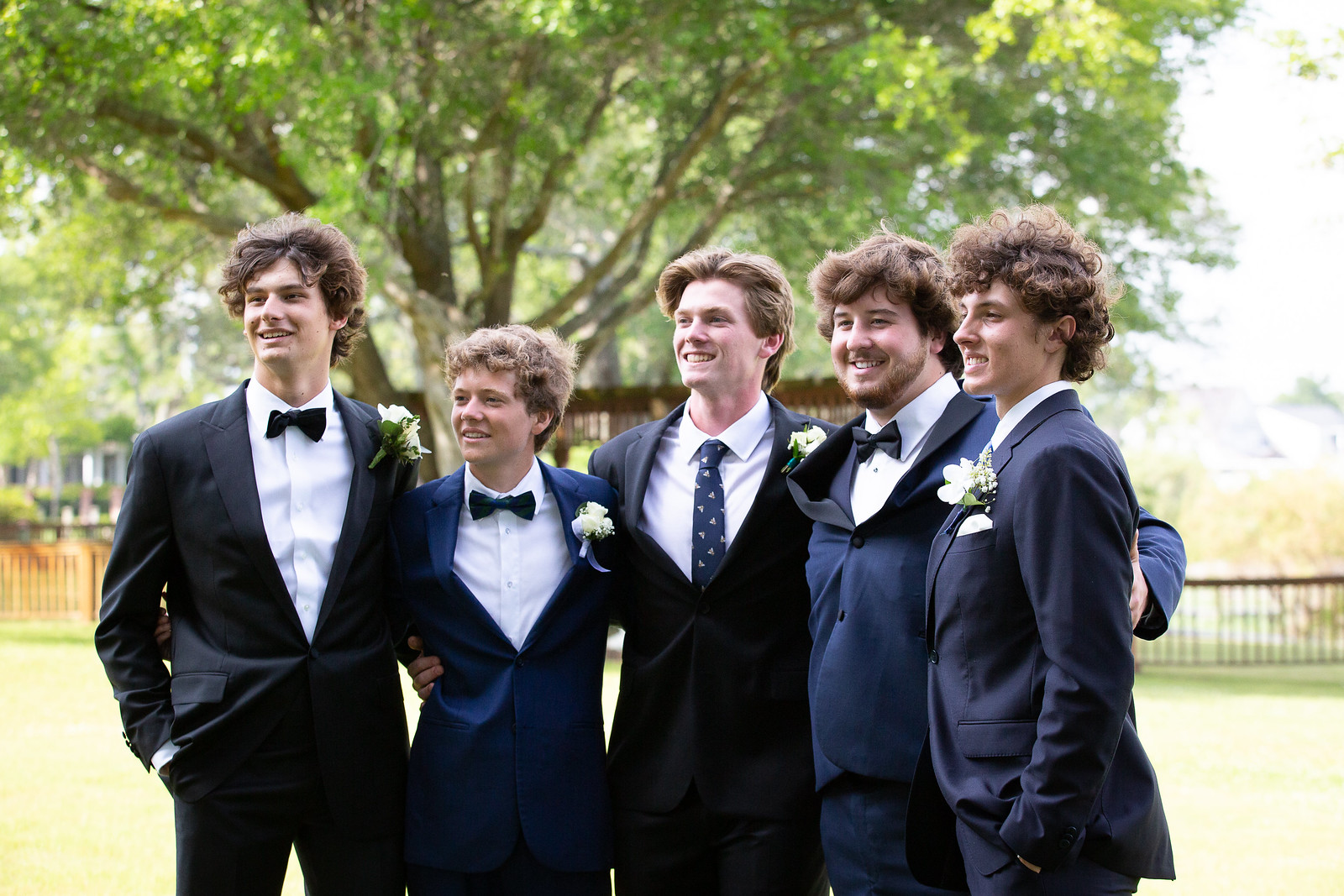The photograph captures a group of five men, likely groomsmen or perhaps including a groom, standing closely together with their arms around each other, dressed in formal attire and posed against an outdoor backdrop. The men are positioned in front of a large tree that spans about three quarters of the image’s width, adorned with bright and dark green leaves. Behind them, a light-colored wooden fence runs along a sunlit lawn with yellow-green grass, basking in bright sunlight.

Starting from the left, the first man is tall with wavy hair, dressed in a black suit jacket and pants, with a white shirt and a black bow tie. His hands are in his pockets, and he wears a white flower corsage on his left lapel. The second man, who is the shortest in the group, is also sporting wavy hair and a blue suit jacket with matching pants, a blue bow tie, and a white shirt. The third man, standing centrally, has wavy hair and a broader smile showing his teeth. He is distinguished by his black suit jacket and a long blue tie featuring a triangle pattern, along with a white shirt and a white flower on his lapel. The fourth man dons a blue suit jacket and pants combination, accented by a black bow tie. The final man on the far right, recognized by his curly hair, is dressed in a navy blue suit jacket and pants, a white shirt, and has his hands in his pockets. Each man wears a white flower on the front flap of their jacket, adding a cohesive and elegant touch to their ensemble.

In summary, the image depicts a closely-knit group of formally dressed men, posed naturally in a serene outdoor setting marked by vibrant foliage and a sunlit lawn.